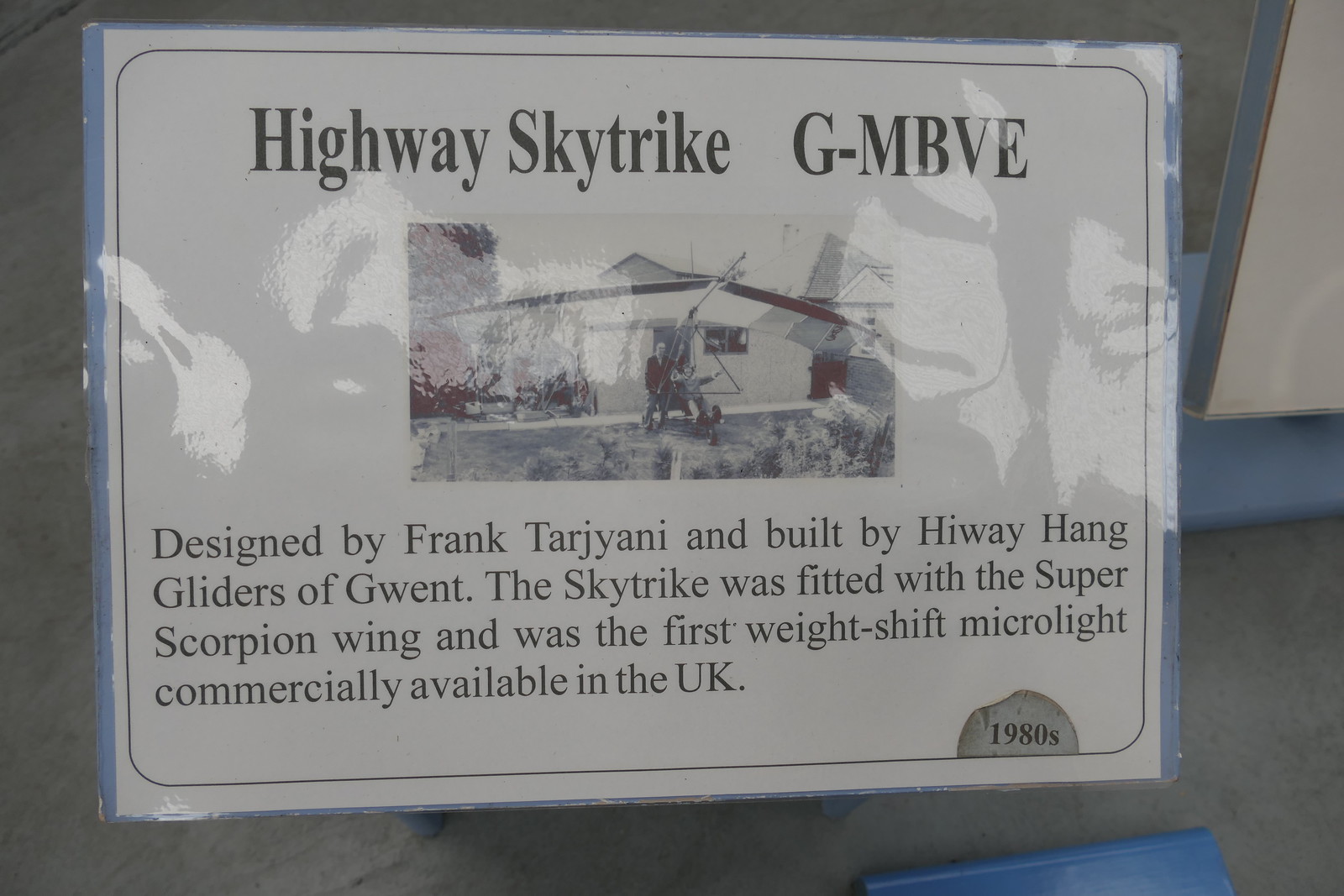This color photograph captures a close-up of an informational sign, which appears to be laminated or possibly behind glass. Mounted on a surface, it features a blue border and is set against a background that includes a concrete or stone floor. The centerpiece of the sign is a small black-and-white photograph depicting a tricycle-like flying device with large wings, known as the Highway Skytrike G-MBVE. The image shows a man standing alone on a front lawn next to this unique vehicle, with a one-story house featuring a sliding window in the background.

The text on the sign reads "Highway Skytrike G-MBVE" at the top, and beneath the photograph, it states, "Designed by Frank Targiani and built by Highway Hang Gliders of Gwent. The Skytrike was fitted with the Super Scorpion wing and was the first weight-shift micro light commercially available in the UK." The bottom right corner of the sign notes that this information pertains to the 1980s.